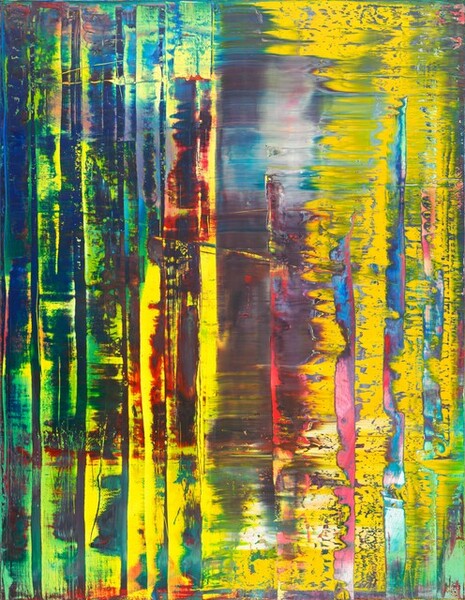The image is a vibrant, monochrome print that appears to be an abstract painting created through a silkscreen process. The dominant color is yellow, with additional hues of blue, green, red, pink, and a purplish blue that blend together to create a psychedelic, almost neon effect. The composition features vertical strokes that run from the top to the bottom of the image, giving the impression of tall buildings or continuous lines that may have been intentionally blurred to create an out-of-focus look. These vertical elements are interspersed with horizontal scrapes, resulting in a dynamic blend of colors and textures. The painting has no discernible objects or text and emphasizes a sense of movement and vivid color interaction, creating an impression of a lively, albeit chaotic urban landscape.